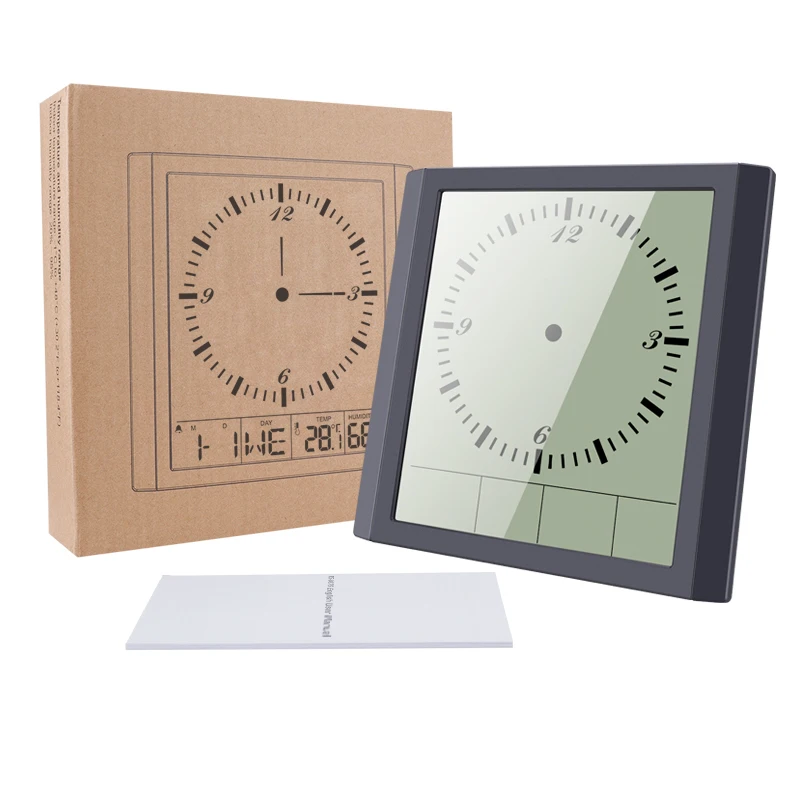This image presents a high-resolution studio photograph likely meant for catalog display, showcasing a digital clock designed in the style of an old analog clock. The clock features a traditional dial with digital hands that simulate analog movement, pointing to the numbered positions at 12, 3, 6, and 9, although the hands are currently not visible on the digital screen. Below the main face, there are four black sub-sections which can display additional information such as the day of the week, temperature, month, and day, akin to a calendar. 

To the left of the clock is the product's package, displayed standing upright. The cardboard box features an image of the digital clock and provides further details, including the clock's multifunctional capacities labeled as W-E, 28, and 68 on its lower part. In front of both the clock and its packaging lies a small, flat pamphlet, presumably an instruction manual, which contains essential setup information for the clock.

All elements are set against a clear white background, providing a clean and focused presentation of the product for potential buyers.